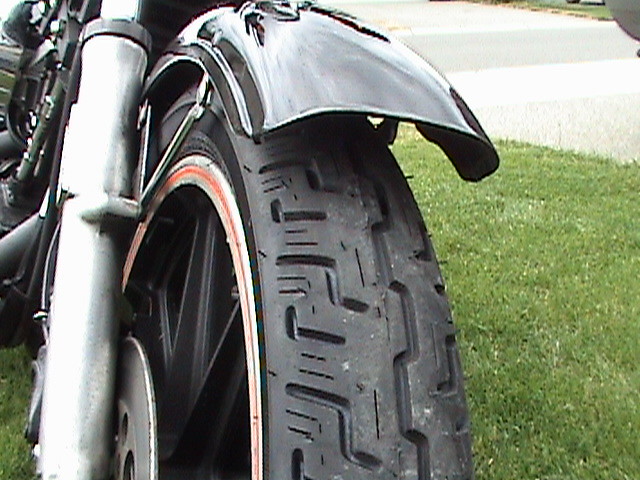This photograph is a detailed close-up of a motorcycle's rear tire set against a grassy background. The tire is black with a distinctive white and orange (or red) stripe running around the sidewall. The primary focus is on the tire itself, particularly the worn tread which features deep, jagged patterns. Above the tire, the black fender is visible, along with the silver struts and shocks extending beside and partially in front of the tire. On the left side of the image, a silver cylinder and part of the motorcycle's side are apparent, though specific details are unclear. Grass occupies the right lower section of the photo, while in the top portion, a small section of pavement or sidewalk is visible, possibly accompanied by a faint, indistinct mark that could be another vehicle. The overall composition highlights the motorcycle's mechanical details against the natural green of the grass and the distant grey pavement.